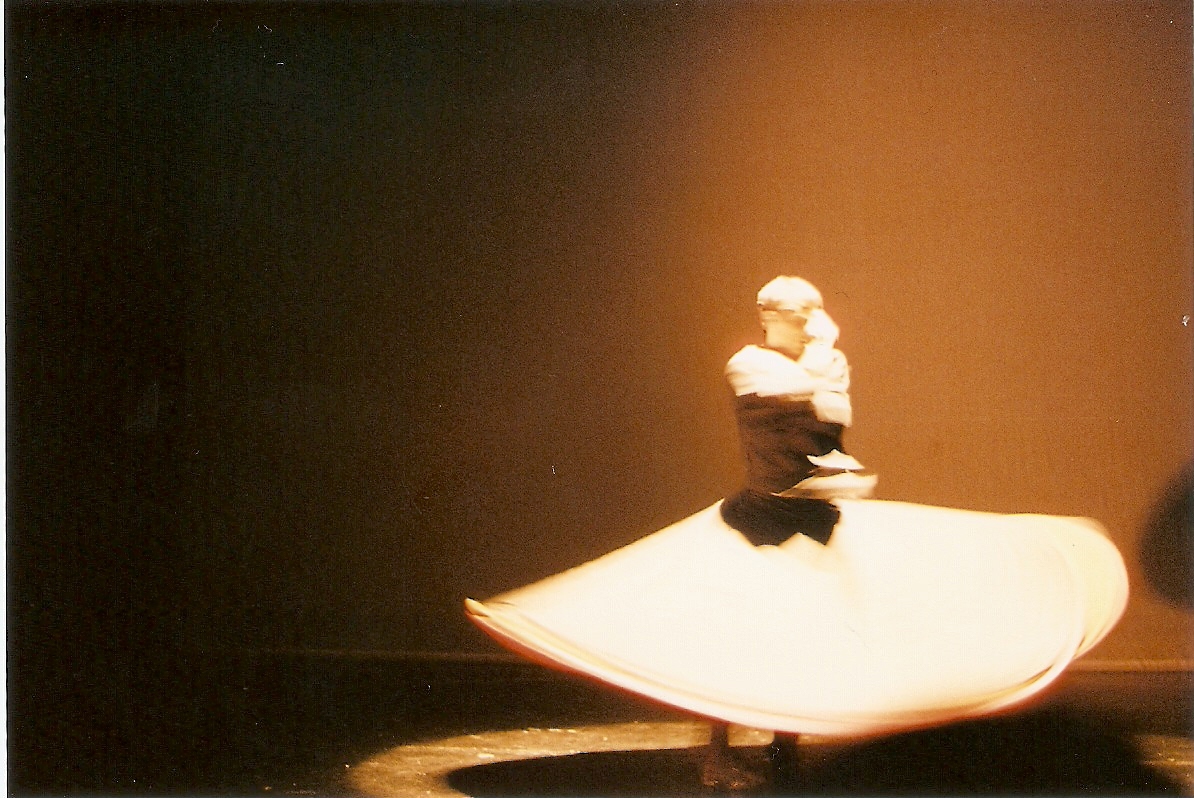The image depicts a detailed sculpture or monument situated on a tan surface with an orangey-brown to dark brown gradient background. The figure, which could represent a woman or a man with short hair, is captured in motion, seemingly dancing or twirling. The lower portion of the figure features a large, white, swirling dress or skirt that extends outward, resembling the shape of an umbrella or a half-pancake. This flowing garment creates a shadow on the floor below. Above the dress, the figure's right hand is raised, possibly near the head or face, while the left hand sits closer to the chest. The blouse or upper attire of the figure is also white or dark brown, contributing to the shadowy play on the dress underneath. The sculpture is highlighted by a white ring of light that seems to reflect around its base, adding to the vibrant detailing of the scene. The setting appears to be indoors, and the figure is oriented towards the right of the photo, adding a dynamic sense of movement.